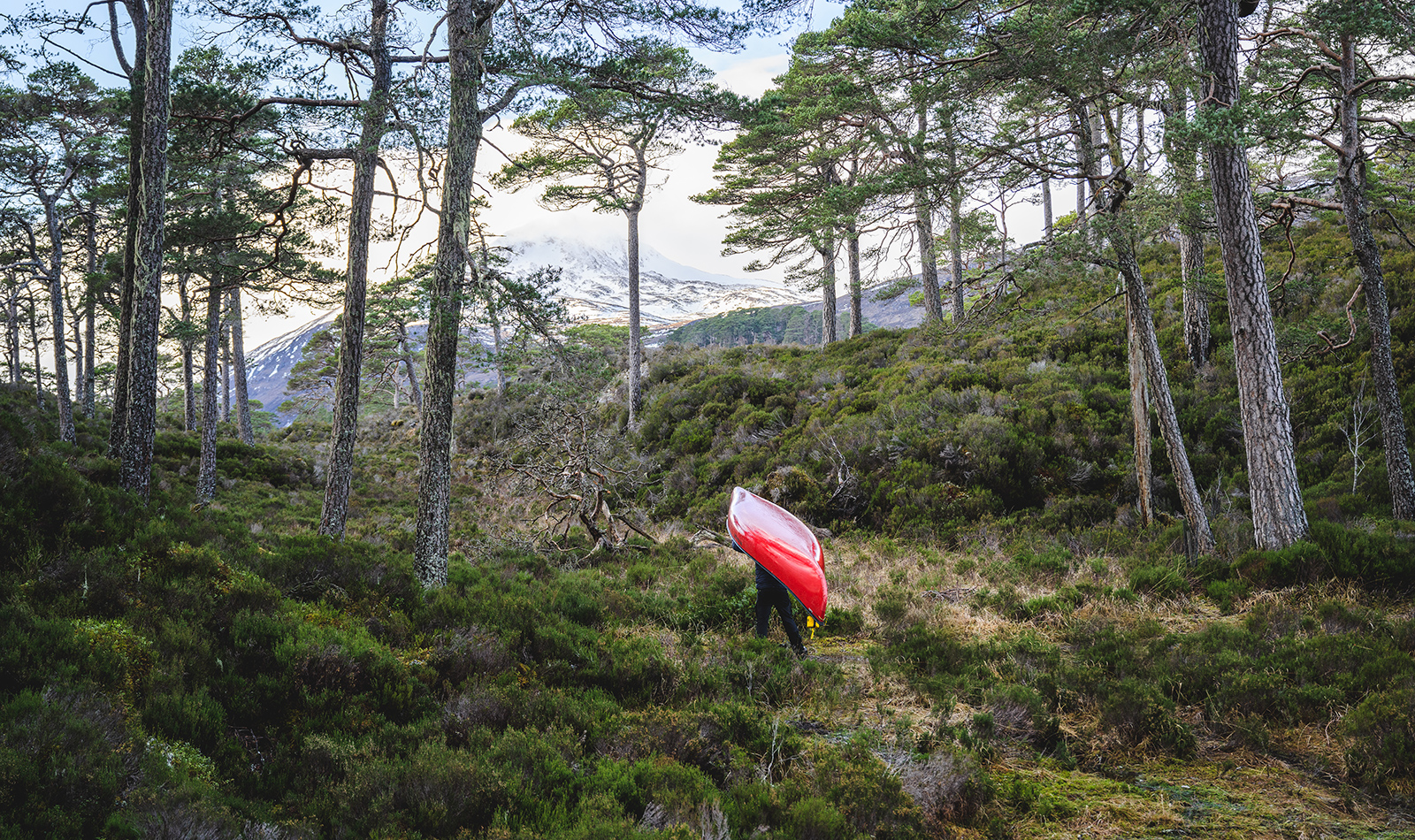In this image, a man is portaging a vibrant red fiberglass canoe through a lush, dense forest. The forest floor is alive with a mix of green leafy plants, tall grasses, shrubs, and patches of light green neon moss, interspersed with some brown and beige vegetation, along with dead branches scattered around. The foliage predominantly comprises big green bushes, creating a puffy green landscape. The trees, mostly cedar with their tall, dark trunks covered in scaly bark, provide a structured canopy overhead. The man, partially obscured by the canoe, appears to be walking through a narrow valley formed by slightly sloped hills on either side, rich with dense underbrush. In the background, a majestic mountain peak covered in snow rises against a backdrop of clear blue skies and scattered white clouds. His journey seems aimed towards this distant and tranquil mountain range.